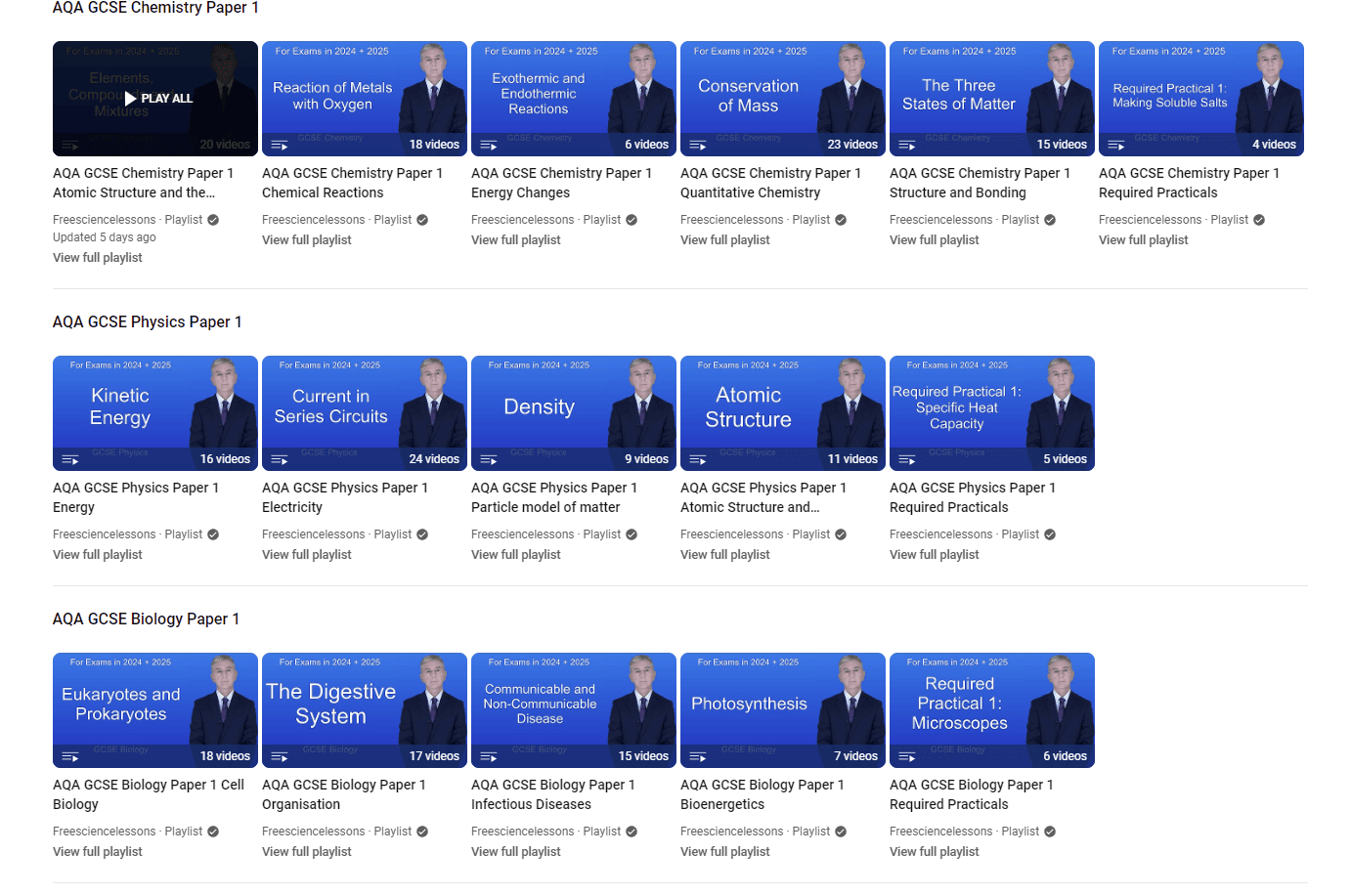This image is a cropped screenshot of a YouTube page, specifically showcasing playlists from the channel "Free Science Lessons". Although the URL or any browser interface elements are not visible, the layout and design unmistakably indicate it’s a YouTube page. 

The screenshot presents three main playlist sections for AQA GCSE examinations, each dedicated to a different subject area: 

1. **AQA GCSE Chemistry Paper 1**: This section displays six playlists. The first playlist's thumbnail features a blacked-out image with a "Play All" button, while the other thumbnails in this section maintain a consistent design—a solid blue background with a photo of a man in a suit on the right, and white text specifying the video's title or subject matter on the left. Playlist video counts range from 4 to 23.

2. **AQA GCSE Physics Paper 1**: Contains five curated playlists following the same visual style as the Chemistry section. Each playlist comprises multiple videos, again with counts varying between 4 and 23.

3. **AQA GCSE Biology Paper 1**: Showcases five playlists, also designed with the uniform blue background and the suited man's image, and white text detailing the video contents. Similar to the other sections, the number of videos within each playlist spans from 4 to 23.

The consistent layout and visual design across all the playlists suggest a cohesive and methodical approach to organizing educational content on the "Free Science Lessons" YouTube channel.